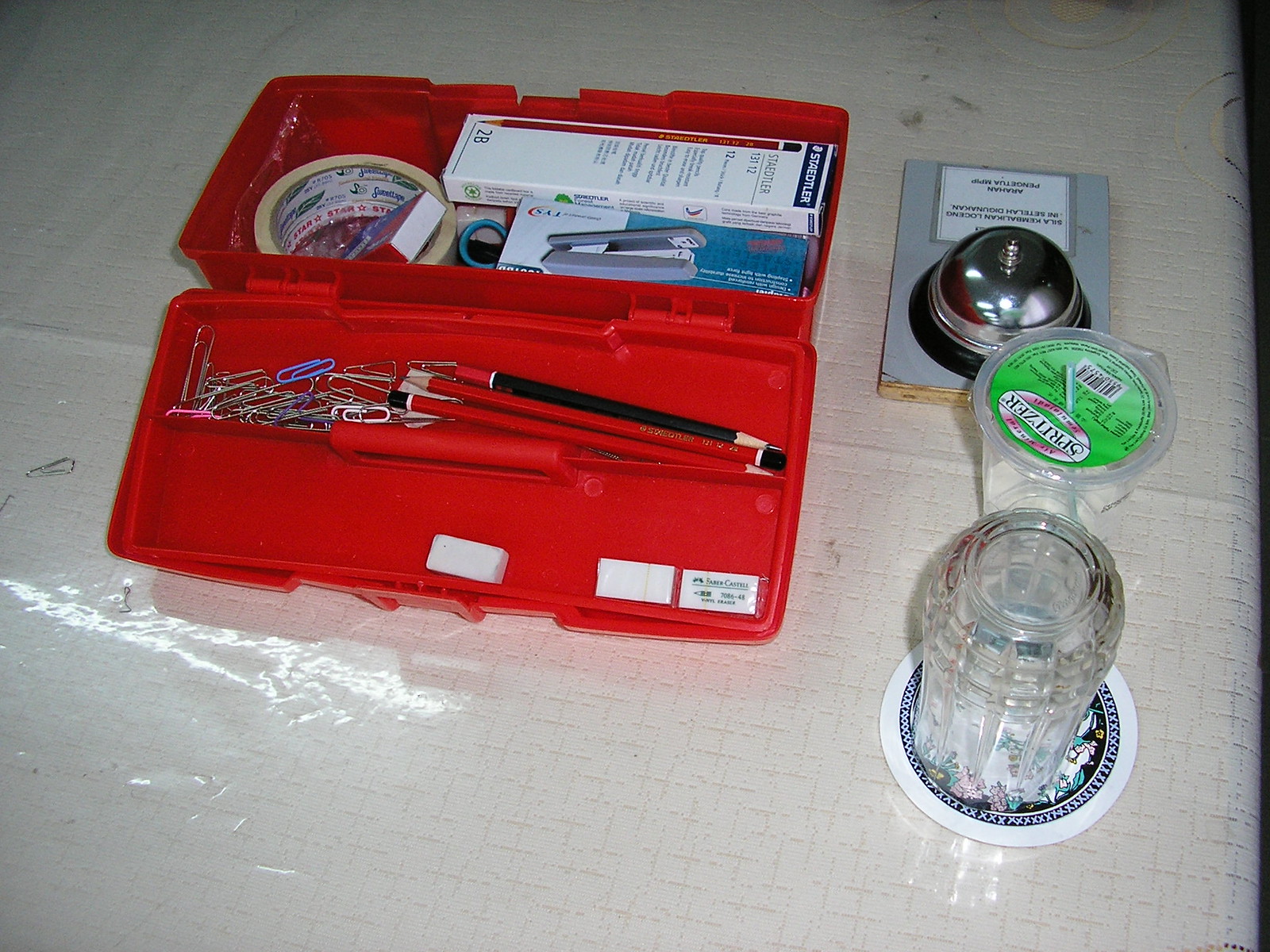The photograph showcases a collection of various items arranged on a white tablecloth, which features faint gold lines. On the right-hand side, there is a white coaster with a blue border adorned with small white X patterns. A glass, turned upside down, partially obscures a subtle floral design on the coaster. Behind this, a clear plastic container with a green "Spritzer" sticker on the lid is visible. Further back, a rectangular piece of wood painted gray serves as a base for a silver bell, the type typically seen at hotel desks, with a black rubber ring around its base. To the left, a red plastic toolbox with a latching lid holds several items, including white erasers, red and black pencils, and an assortment of silver, white, and blue paper clips in its inner tray. Inside the box, you can also spot red 2B-labeled pencils, a gray stapler, blue scissor handles, masking tape, and staples.